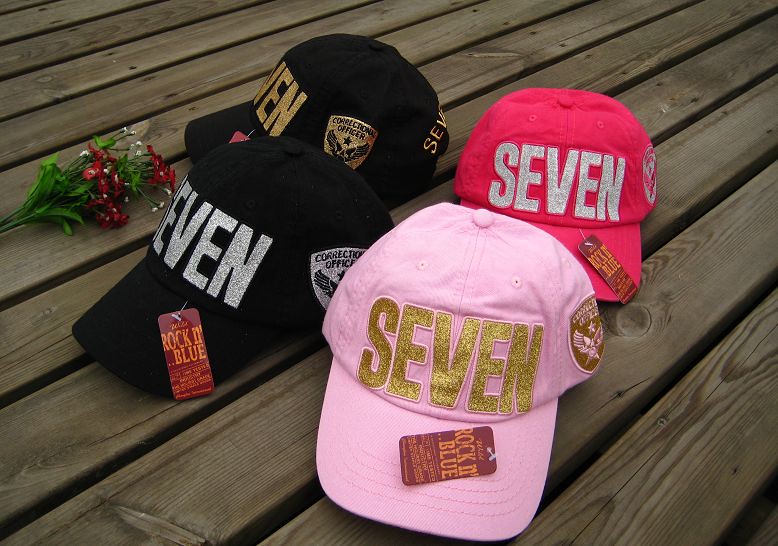This is a landscape-oriented photograph showcasing four baseball caps displayed on a timber deck made of diagonally-arranged brown wooden planks with light brown accents. The caps, which are stylistically identical but vary in color, each feature the word "SEVEN" prominently on the front. Two of the caps are black, one with silver lettering and a side badge featuring an eagle and the words "CORRECTION OFFICER" in silver, and the other with gold lettering and a corresponding gold badge. Another cap is light pink with gold lettering and a gold badge, while the final cap is a bright pink with silver lettering and a silver badge. All caps also have paper tags attached with plastic strings that read "ROCK THE BLUE." Adjacent to the caps, on the left side of the image, sits a green-stemmed plant with green leaves and a bouquet of red flowers with white centers.